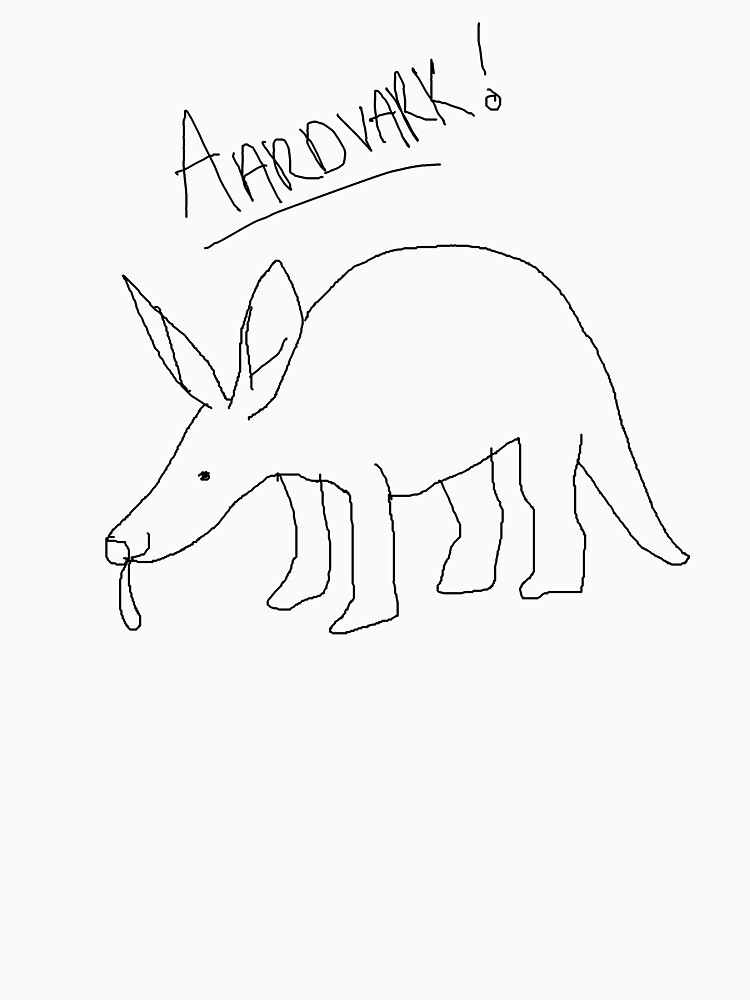This image showcases a hand-drawn illustration of an aardvark on a piece of white paper. At the top, angled slightly toward the upper right, the word "AARDVARK" is prominently written in bold, capital letters and underlined, with an exclamation point for emphasis. Below this text, which appears to be done with a marker or pen, is the main drawing of the aardvark. The animal is depicted in a childlike, black-and-white outline style. 

The aardvark is presented from a left side view, featuring a single visible eye drawn as a small black dot. Its long ears stand upright and slightly outward, while its snout points left with a distinctly long, teardrop-shaped tongue that sticks out and slopes downwards. The aardvark's back is slightly humped, and it stands on all four legs with a long, wide tail that points down to the ground. The overall appearance suggests a simplistic, whimsical sketch, capturing the essential features of the aardvark in an endearing and straightforward manner.